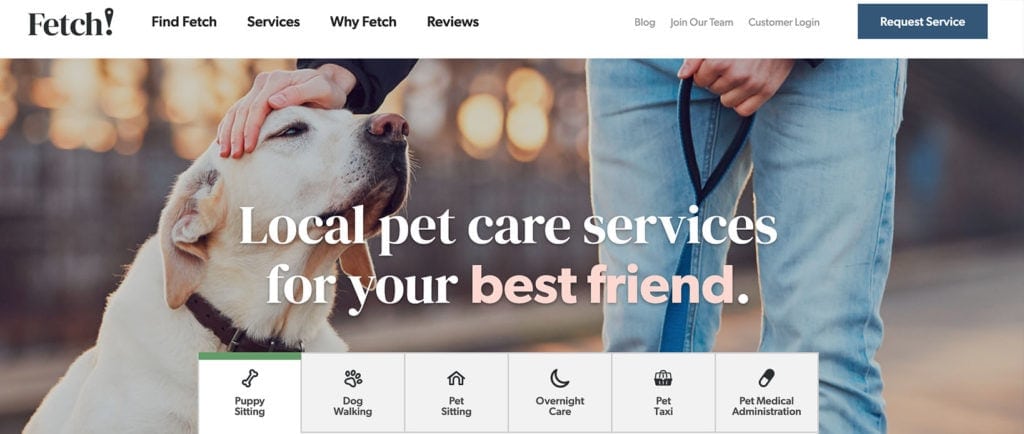Screenshot of the Fetch website interface. 

In the top left corner, there's the Fetch logo, distinguished by an exclamation mark. Adjacent to the logo, the navigation bar includes the following sections: `Find Fetch`, `Services`, `Why Fetch`, and `Reviews`. On the top right, a line of gray text appears too faint to decipher, alongside a prominent dark blue button labeled `Request Service` in white font. 

Below this navigation bar, the main header section features a wide, horizontal image capturing an affectionate moment between a dog and a person. On the left side of the image is a close-up of a dog's face with a hand gently resting on its head. To the right, part of a person's legs is visible, holding a leash. The backdrop includes a street scene with blurred lights, adding depth and context to the scene. 

Centrally positioned over the image, bold white text reads: "Local Pet Care Services for Your Best Friend," with the words "best friend" emphasized. 

A white rectangular overlay at the bottom of the image displays six horizontally aligned icons: a bone, a paw print, a house, a moon, an indeterminate icon, and a pill. Each icon is accompanied by small text that is unreadable due to its size.